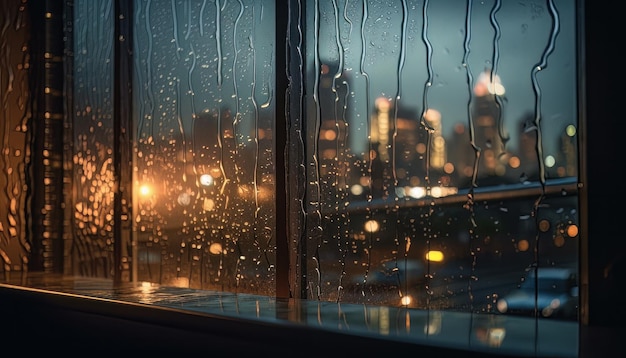This detailed image showcases a nighttime urban scene viewed through rain-speckled window panes. At the forefront, the reflective surface of a window with multiple panes, bordered by brown and lighter brown casings, dominates the composition. The window structure includes vertical and horizontal elements, which create an intricate pattern against the dark backdrop. Rain droplets are clearly visible on the glass, enhancing the window's shiny, black coating.

Beyond the window, though slightly blurred, you can discern a city skyline illuminated by various lights, with buildings stretching into the distance under a grayish-blue sky. In the bottom right, there are cars traveling on a street, their headlights contributing to the multitude of lights reflected on the wet glass. Notably, there seems to be a bridge or railway cutting across the scene from left to right. The color palette of the image comprises blues, blacks, whites, and yellows, creating a visually striking and aesthetically pleasing night scene, depicted from the perspective of someone looking out from inside a cozy space.